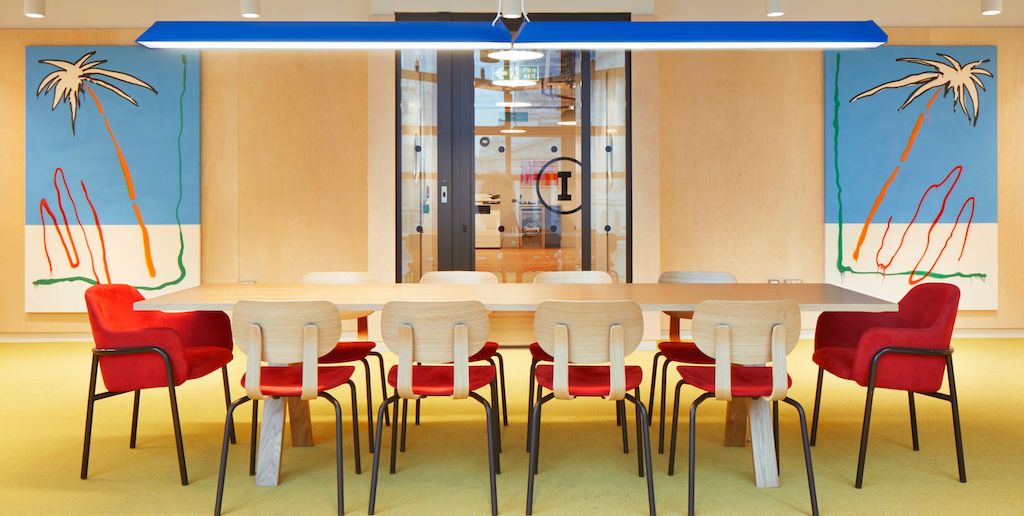This indoor image is a 3D color illustration, likely created using an application such as SketchUp. The composition is in landscape orientation and depicts a meeting space with a long rectangular conference table that has a beige, wood-like surface and a peach-colored tabletop. The table is flanked by 10 chairs, with one chair at each end and four chairs along each side. The end chairs have orange seats with black metal frames, while the side chairs feature white backs and orange seats mounted on black metal legs.

The floor is a light lemon yellow shade, and the walls around the space are a peach color. Hanging above the table is a bright blue, pendant-style light fixture as wide as the table itself, illuminating the space below. On the back wall, there are two pieces of abstract wall art featuring simply drawn palm trees with blue tops and white bottoms, accompanied by red and green squiggly lines. One palm tree faces right on the right side, and the other faces left on the left side. The artwork is unframed and minimalist in design.

A door situated underneath the light fixture opens into another room, hinting at the office setting of the space.